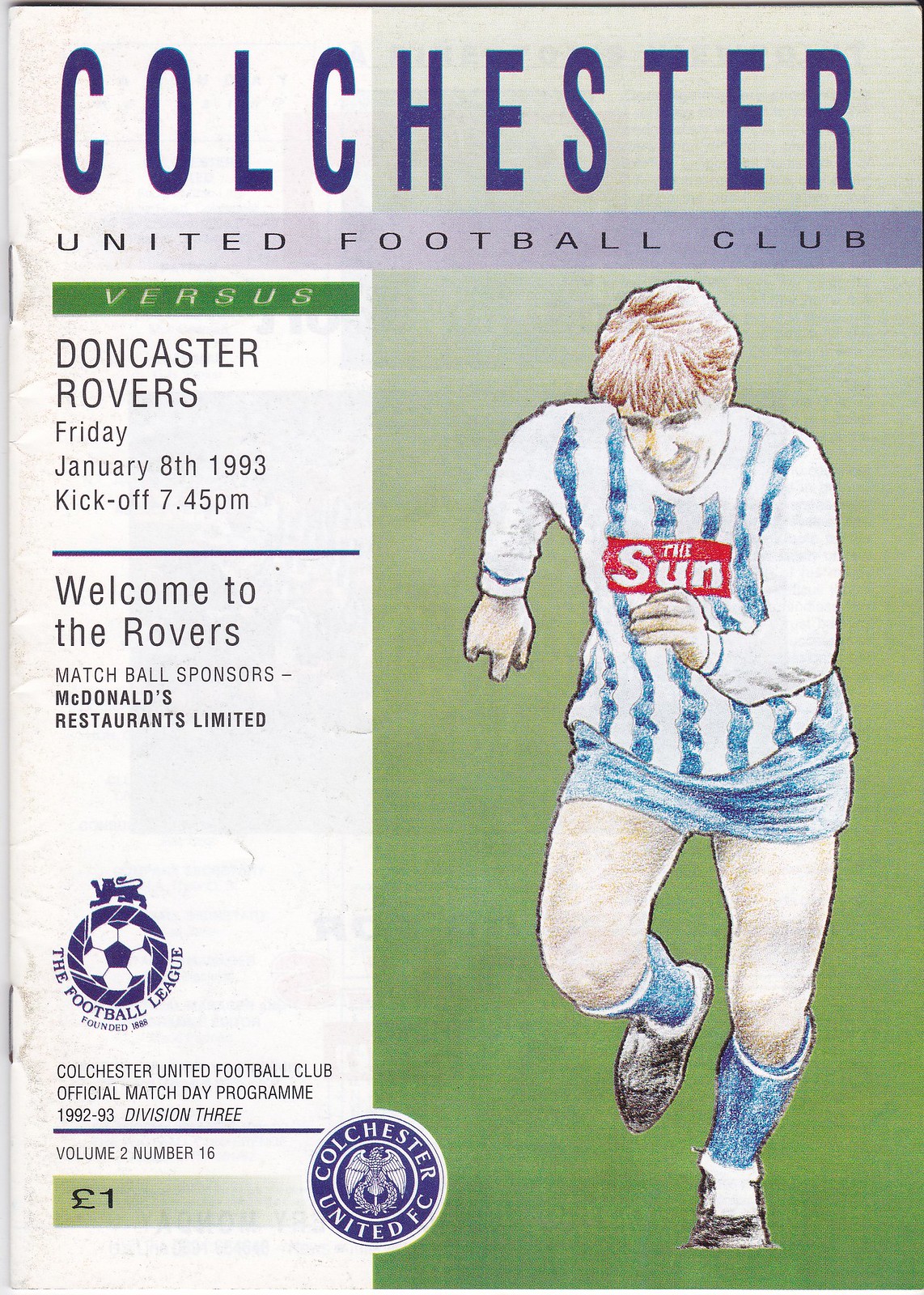This image is the cover of a sports program for a soccer match between Colchester United Football Club and Doncaster Rovers, scheduled for Friday, January 8th, 1993, with a kickoff at 7:45 p.m. At the top in prominent purple letters, it reads "Colchester United Football Club." The main visual element is a caricature of a soccer player with light or possibly reddish hair, running head-down toward the viewer on a green field. He is dressed in a blue and white vertically striped jersey, blue shorts, blue socks, and black shoes. The jersey features a red rectangular logo with the word "SUN" in white letters. Additional text on the cover includes "versus Doncaster Rovers," along with the match details and sponsor information mentioning McDonald's Restaurants Limited. Towards the bottom, there is a logo featuring a globe with a soccer theme and a lion on top, representing the Football League, and another logo for Colchester United FC Football Club. On the bottom left, there's a faded green box indicating that the entrance ticket is priced at one euro.